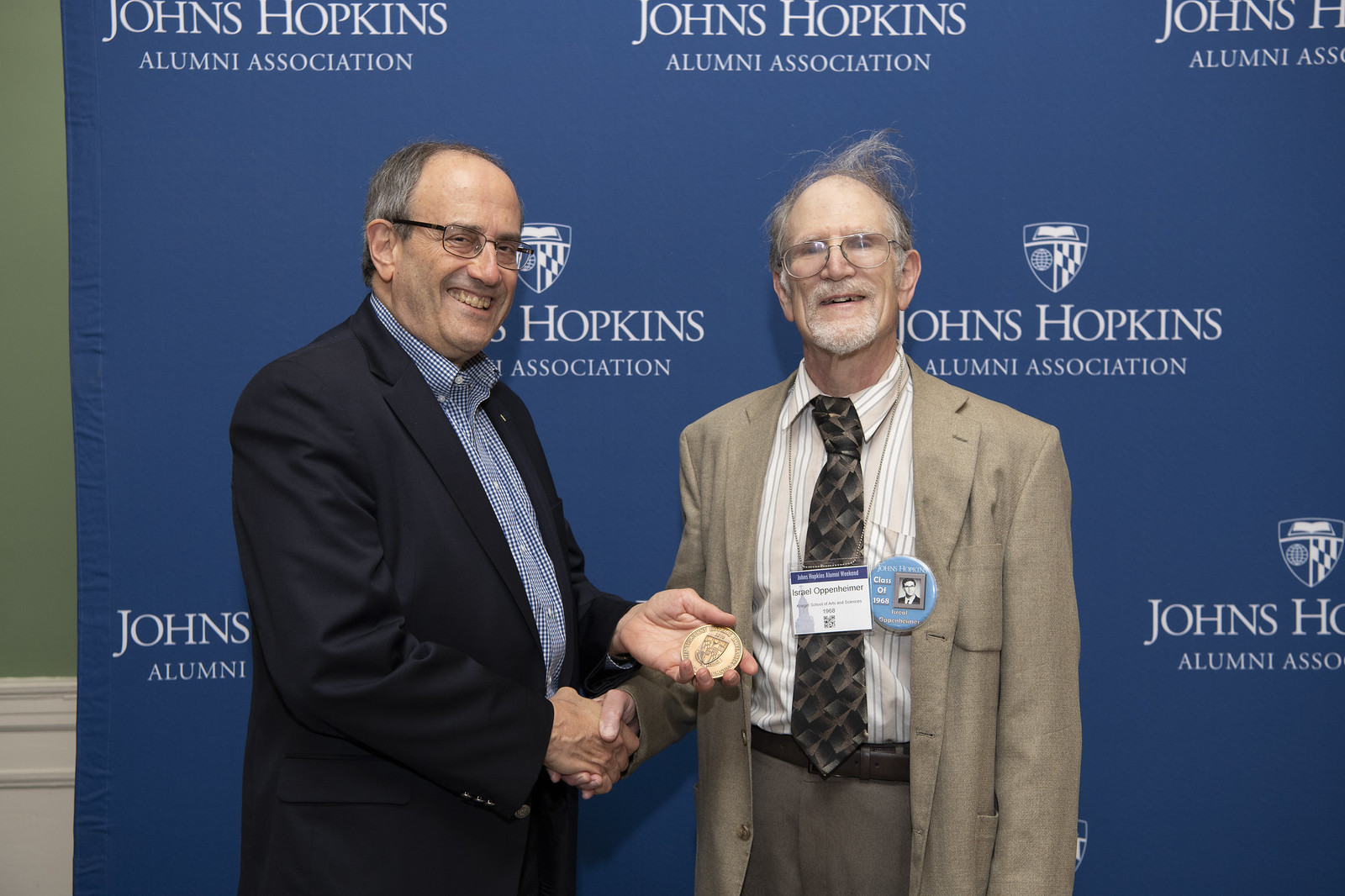The photograph features two men standing in front of a blue banner adorned with the Johns Hopkins Alumni Association logos. The partial view of the background reveals a green wall with a white bottom section on the left side of the image. The man on the left is dressed in a black suit jacket and a blue button-up shirt, complemented by black-framed glasses. He is shaking hands with the man on the right and holding a large, gold medal in his left hand. The older man on the right has a distinctive look with his messy gray hair and beard. He is wearing a light brown suit, a grayish-brown tie with a diamond pattern, gray pants, and a brown belt. His attire also includes a white and tan-colored striped shirt. Their interaction suggests a moment of recognition or celebration related to the Johns Hopkins Alumni Association.